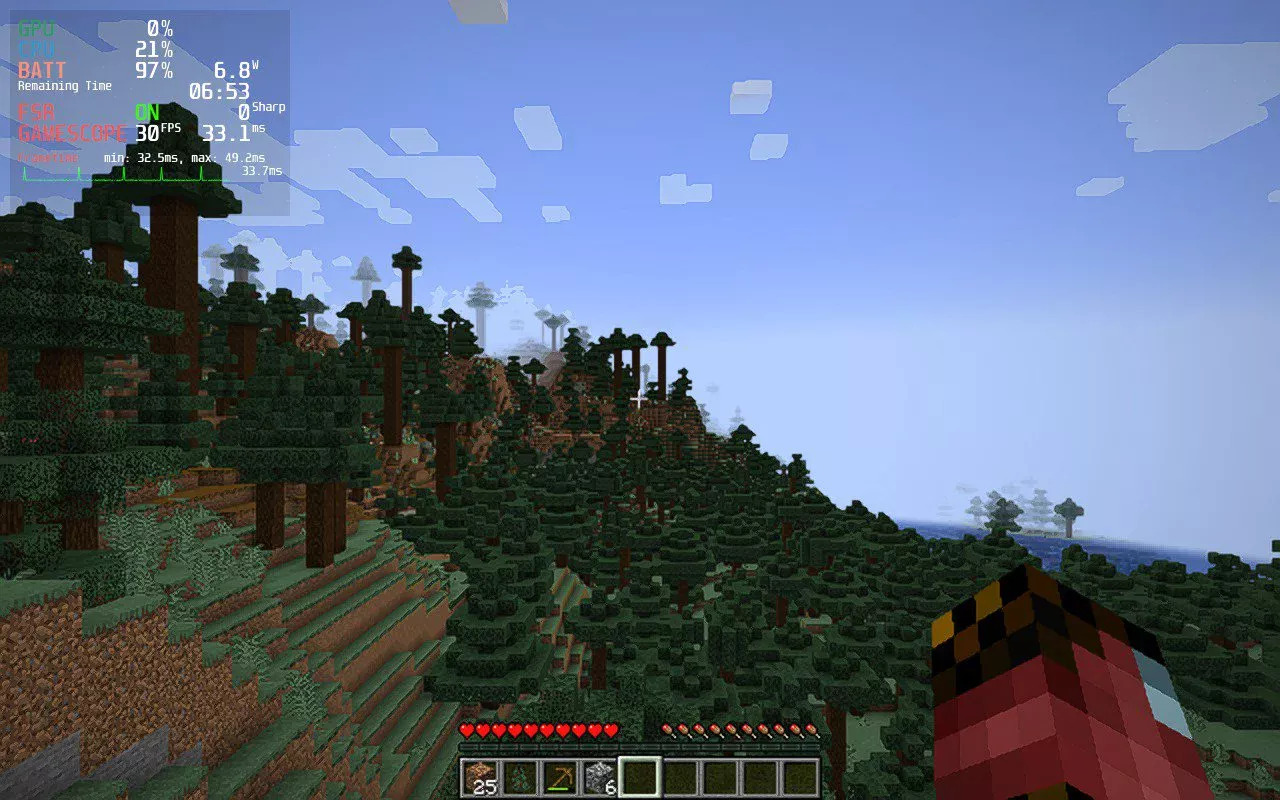The image is a screenshot from the game Minecraft, featuring a player’s point of view. In the foreground, at the bottom center of the screen, there's a row of gray item slots. The first slot on the left contains the number '6' in white, the second slot has the number '25' inside a brown square, symbolizing an item quantity. To the right of these numbers, there's an icon of a tree in another slot, followed by a green and brown tool, presumably a shovel or pickaxe. Above these item slots, on the left side, red heart icons indicate the player’s health. On the right side above the slots, there are red, brown, and white shapes resembling other icons or items.

The landscape displays a hill inclined from the top left to bottom right, populated with blocky trees having green leaves and brown trunks. The hill’s formation gives a step-like appearance, typical of Minecraft's block-based graphics. There are some mountain shapes in the background with a mixture of green grass, brown soil, and occasional gray rocks. The sky is bright blue with square white clouds scattered throughout. On the bottom right, there is a section of an ocean visible.

Additionally, overlaying the top left of the screen is a transparent square showing performance metrics in various colors such as green, blue, orange, white, and red. It details information like GPU usage at 0%, CPU usage at 29%, battery at 97%, and various timing and performance statistics.